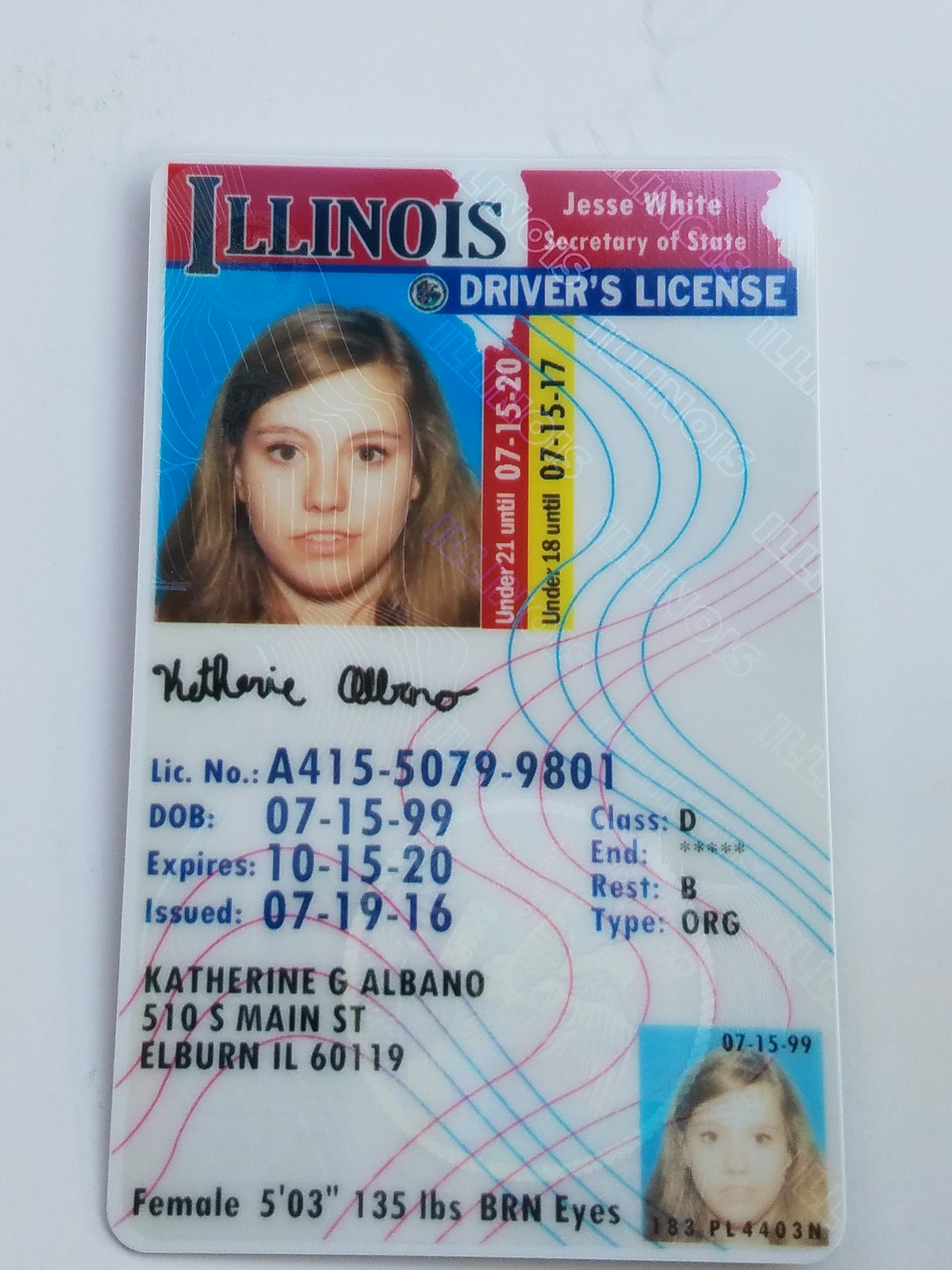The image depicts a driver's license belonging to a woman named Catherine G. Albano. The license, which is placed on a white marble surface, has a distinct appearance with a red border at the top, under which it reads "Illinois, Jesse White, Secretary of State" in black lettering. Below this header, "Driver's License" is written in white letters on a blue background. The left side of the license features a photograph of a young woman with long brown hair, staring directly ahead against a blue background. Adjacent to the photo, written vertically in a red section, are the words "Under 21 until 07-15-2020," and directly below this, in yellow, it states "Under 18 until 07-15-2017." The license also includes Catherine's signature beneath her photograph. Additional details, including her license number (84150-5079-9801), date of birth, expiration date, and issue date, are written in blue letters. At the bottom left, it provides her name and address: Catherine G. Albano, 510 South Main Street, Elburn, Illinois. The license further indicates her personal details—female, 5'3", 135 pounds, with brown eyes. A smaller image of the same photograph appears in the lower right corner of the driver's license.